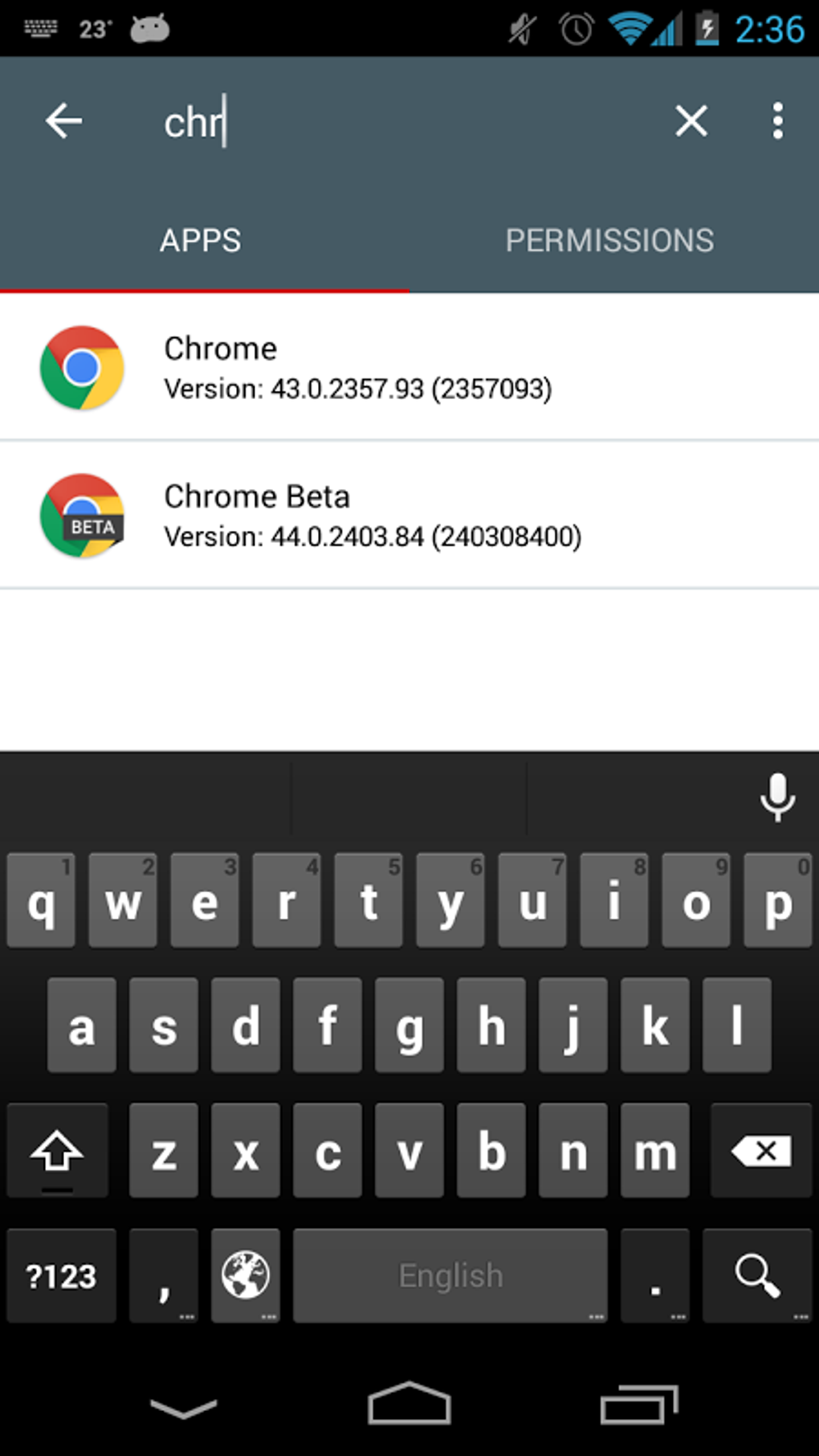In this screenshot, the image captures a search interface with a focus on an application search. At the top, a search bar prominently displays the typed query "CHR." To the left of the input text, a back arrow button allows for navigation to the previous screen, while to the right, there are a close (X) button and a three-dotted menu icon for additional options. Beneath the search bar, two tabs are visible: "Apps" on the left and "Permissions" on the right, indicating the search can be filtered by application types or permissions.

The search results show two entries. The top entry is "Chrome" with the version number 43.0.2357.93, and the entry beneath it is "Chrome Beta" with the version number 44.0.2403.84. Both entries prominently display the Chrome logo to the left of their respective text. Notably, the Chrome Beta entry features a distinctive beta banner overlay at the center of the logo.

The bottom half of the screenshot is occupied by an on-screen keyboard, which includes a microphone symbol located in the top-right corner, hinting at voice input capability. At the very bottom, a black navigation bar spans the width of the screen. This bar includes several icons: an arrow pointing downward, a home symbol, and a button designed to access other tabs or recent applications.